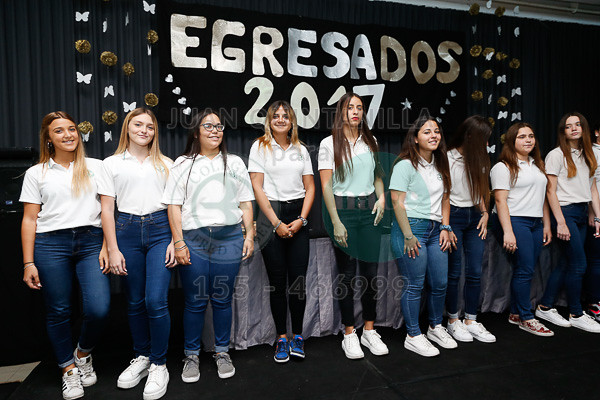The photo captures a lineup of nine young women, possibly graduates, standing in front of a closed curtain adorned with various decorations. The backdrop features the word "Egresados" in prominently cut out letters with '2017' displayed beneath it. The word "Egresa" is in white, "Dos" is in gray, and "2017" is also in white. Diagonal rows of hearts and a star embellish the bottom, alongside stringed decorations resembling butterflies and small, round gold objects, possibly flowers.

All the girls are similarly dressed in white collared t-shirts and jeans, though the center two might be in black jeans due to their positioning behind a partially visible watermark. This faint watermark appears to read "Collegio Alfred Nobel," accompanied by an image of a bird within a circle, and another part showing "n-a-c-e" in pink on a green circle with numbers "155-466-999" beneath it. Footwear varies from predominantly white sneakers to a few in gray, blue, red, and floral designs. The girls, appearing to be preteens or teenagers, display an assortment of blonde, brunette, and black hair, with only one wearing glasses. The photo appears to be taken in a small auditorium or similar space prepared for a celebration or graduation event.